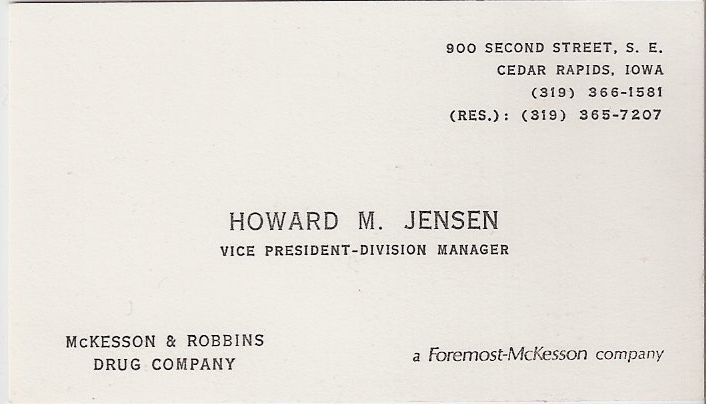The image showcases a plain, white business card featuring black text, conveying essential contact details in a clear, straightforward manner. Centered prominently on the card is the name "Howard M. Jensen" with the titles "Vice President, Division Manager." Positioned in the top right corner, the address reads "900 2nd Street, S.E., Cedar Rapids, Iowa," accompanied by two phone numbers: "319-366-1581" and "Residence: 319-365-7207." The bottom left corner of the card displays the company name "McKeeson & Robbins Drug Company," while the bottom right corner states "A Foremost McKeeson Company." The overall design is minimalistic, ensuring easy readability of the pertinent information.